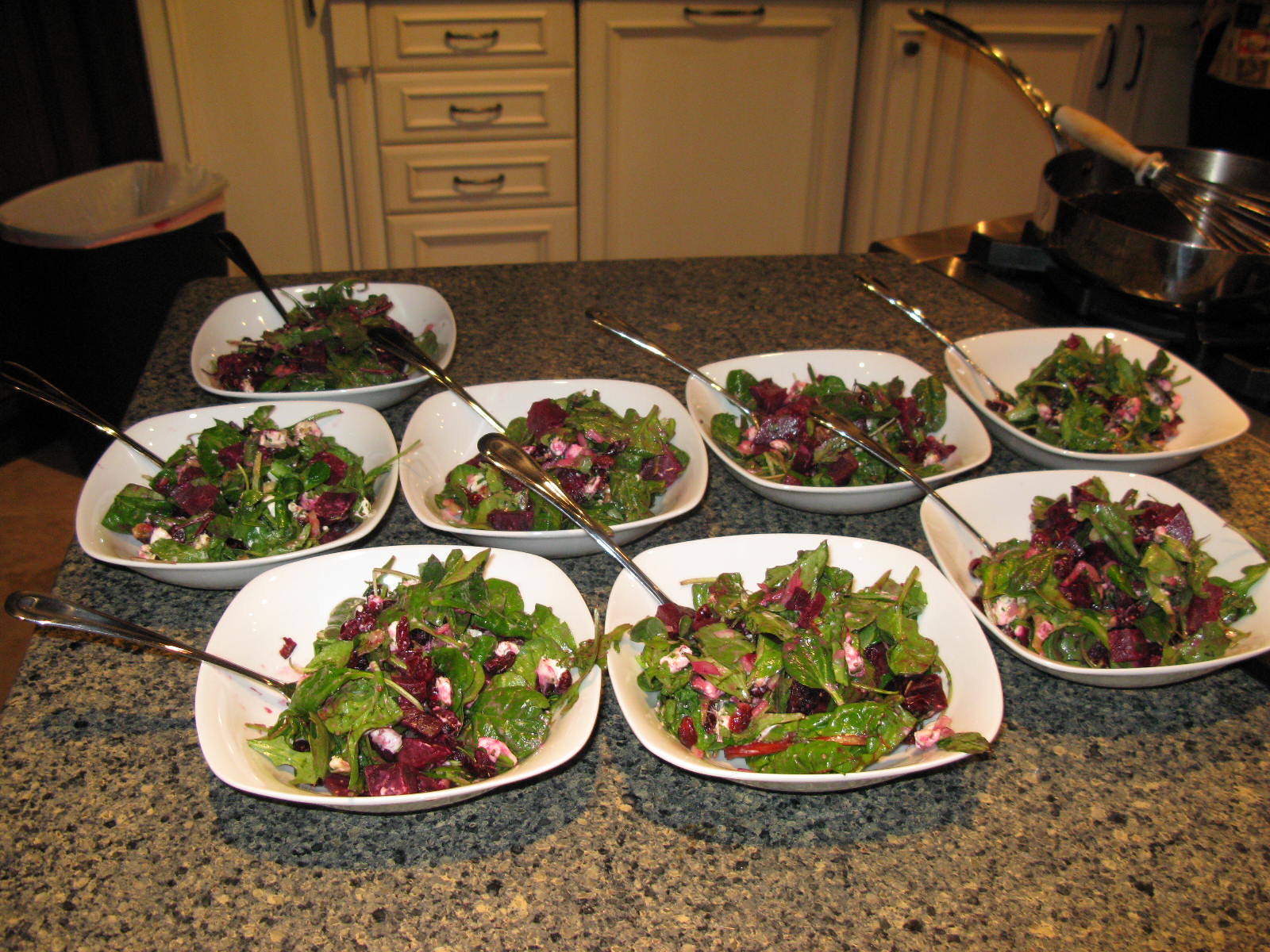In this domestic kitchen scene, we see a granite countertop with a striking design of black, tan, gray, and white resembling paint flakes. On this expansive counter, there are eight white shallow bowls filled with a colorful salad mix. The salad appears to feature baby spinach leaves, possibly some wilted, along with ingredients like chopped beets and small white cheese pieces, and a sheen that suggests the dressing has already been applied. Each bowl has a silver fork placed inside, oriented towards the left. The bowls are arranged with three in the front, four behind them, and one slightly to the left behind the row of four. To the left of the image is a black trash can, while the top right features a stove with a silver pan and a whisk, and a brown handle sticking out. The back area has off-white kitchen cabinets, which include drawers and possibly a fridge. The foreground is brightly lit, transitioning to a darker background, highlighting the various elements of this well-used kitchen space.